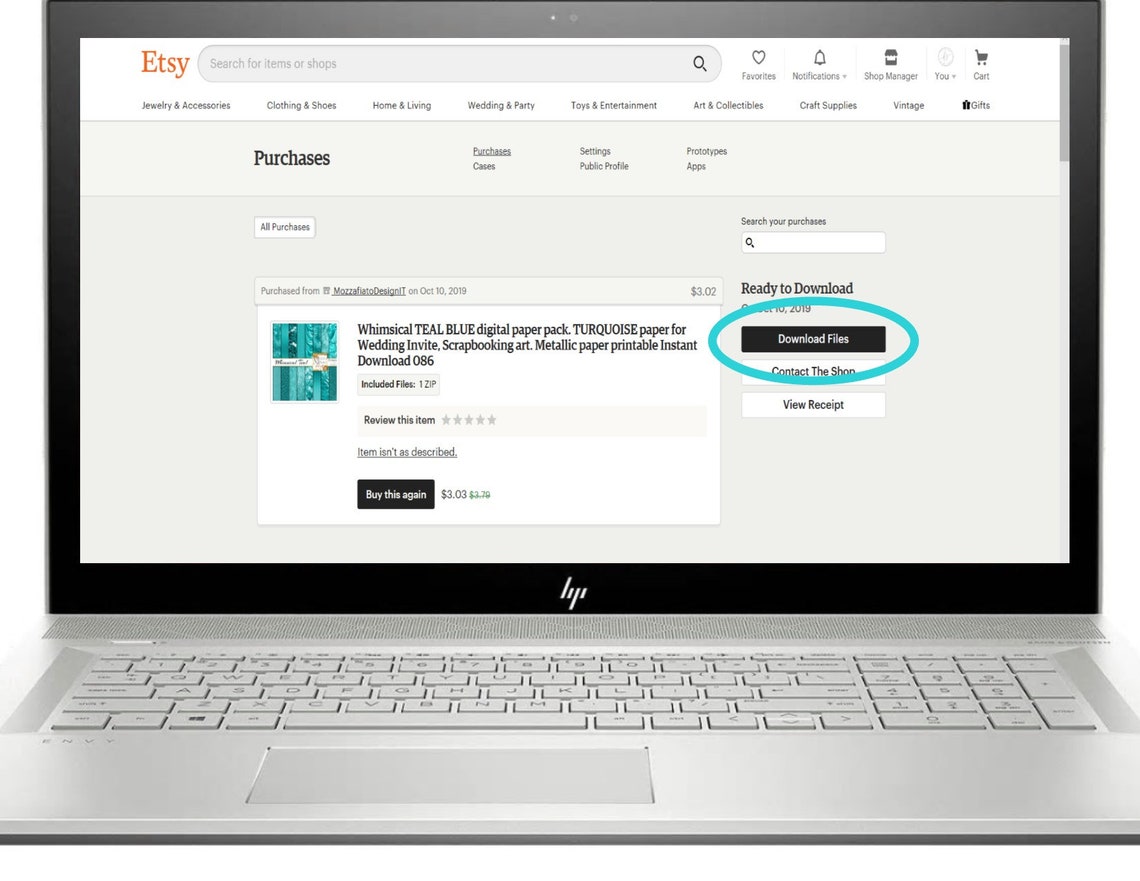The image features an open silver HP laptop prominently displaying the Etsy website. The screen's contents are highly detailed, starting at the top with the Etsy logo in orange letters and navigation options such as "Search for items or shops," "Favorites," "Notifications," "Shop Manager," "You," "Cart," as well as various category links like "Jewelry and Accessories," "Clothing and Shoes," "Home and Living," and more.

In-depth details include specific account information, such as tracked purchases like a "Whimsical Teal Blue Digital Paper Pack" purchased from Matza Fiato Design IT on October 10, 2019. This product is described as "turquoise paper for wedding invites, scrapbooking, metallic paper, printable, instant download 086," and the files included in the purchase come in a zip format. 

Additionally, there are user interaction options such as "Review this item," with "Item isn't as described" underlined, and "Buy this again," next to the listed prices of $3.03 (marked down from $3.79). To the right, the text "Ready to download" and "Download files" is highlighted within a turquoise circle. The screen also offers further options like "Contact Shop" and "View Receipt." The setting appears to be free of any people.